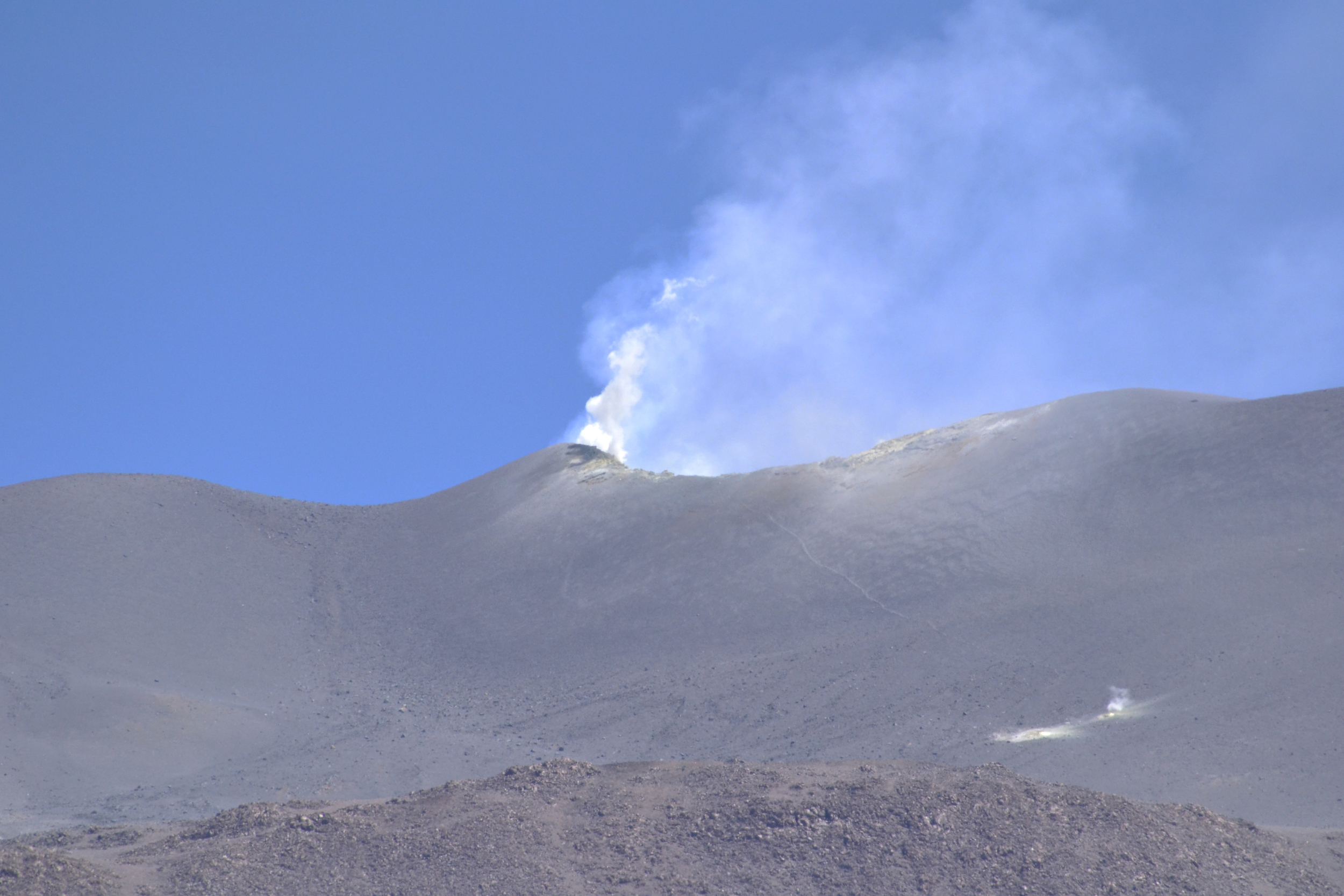The image is a color photograph depicting a desolate, rocky mountainside that is predominantly gray and black, with a landscape that appears smooth yet slightly rocky. A significant feature of the scene is a plume of smoke rising from what seems to be a vent or fissure on the mountain, indicating possible volcanic activity. However, the vent itself is not visible, adding to the mystery. At the bottom of the image, patches of dirt and a small white area, which might be snow or salt, are visible. The scene is set under a vast, bright blue sky taking up the top 40% of the image, while the central portion features the smoky vent, and the lower half is dominated by the barren, earthy terrain. The photograph captures the stark, isolated beauty of a possibly volcanic environment, devoid of foliage or other prominent features, focusing entirely on the raw, unadulterated elements of nature.